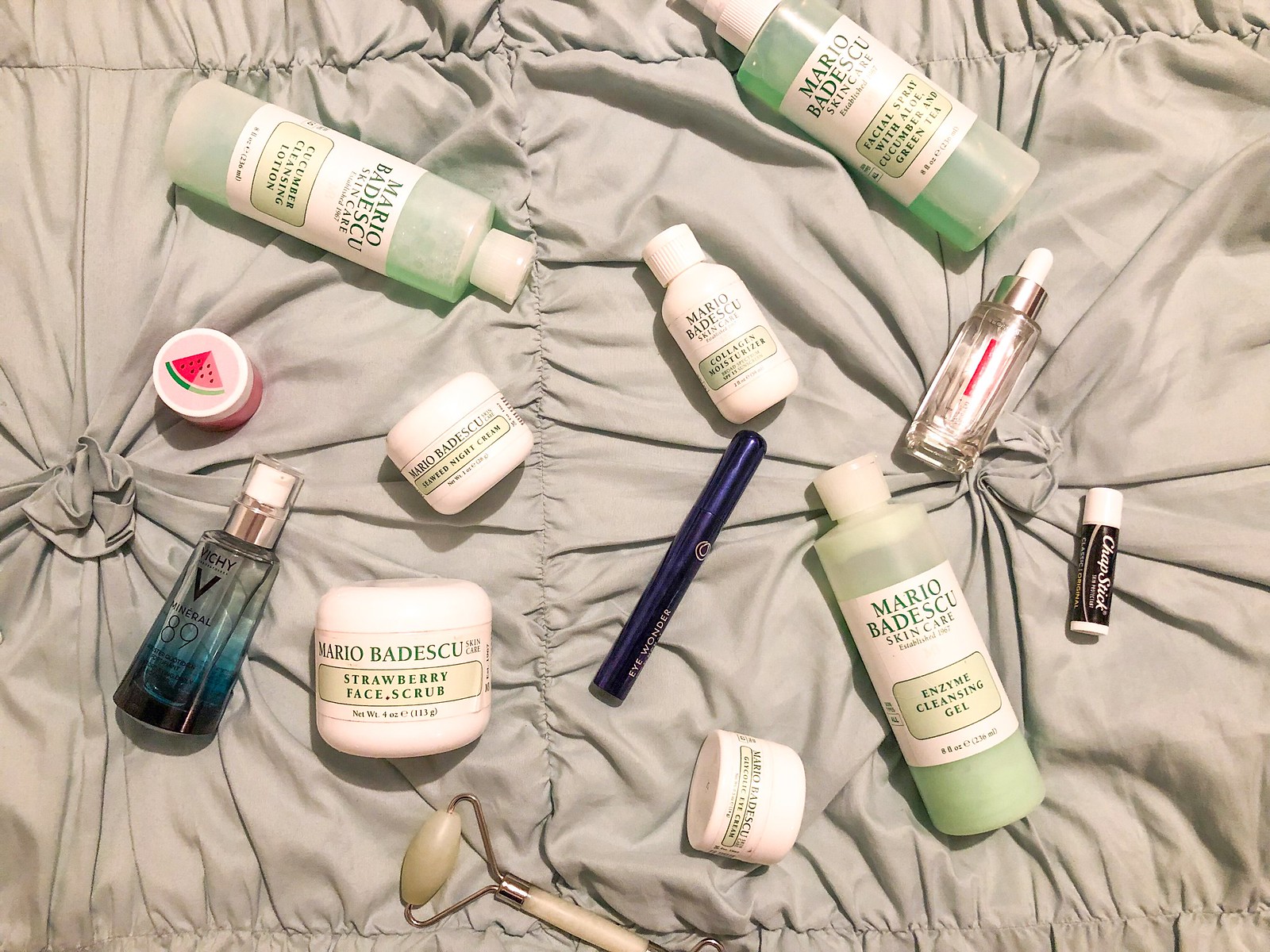A collection of Mario Badescu Skin Care products is meticulously arranged on a tan or beige comforter atop a bed, creating a visually appealing display. Featured prominently are several items, including an enzyme cleansing gel, a strawberry face scrub, a night cream, a collagen moisturizer, a cucumber cleansing lotion, and a facial spray with aloe, cucumber, and green tea. Additionally, a small canister containing another cream by Mario Badescu is present. The scene is complemented by a manual massage tool, likely intended for back massages, along with a tube of chapstick, a mascara, and a mineral product by Vichy. The Vichy bottle, distinct with its clear design and blue-tinted bottom, adds a touch of elegance to the diverse assortment of skincare and beauty products.